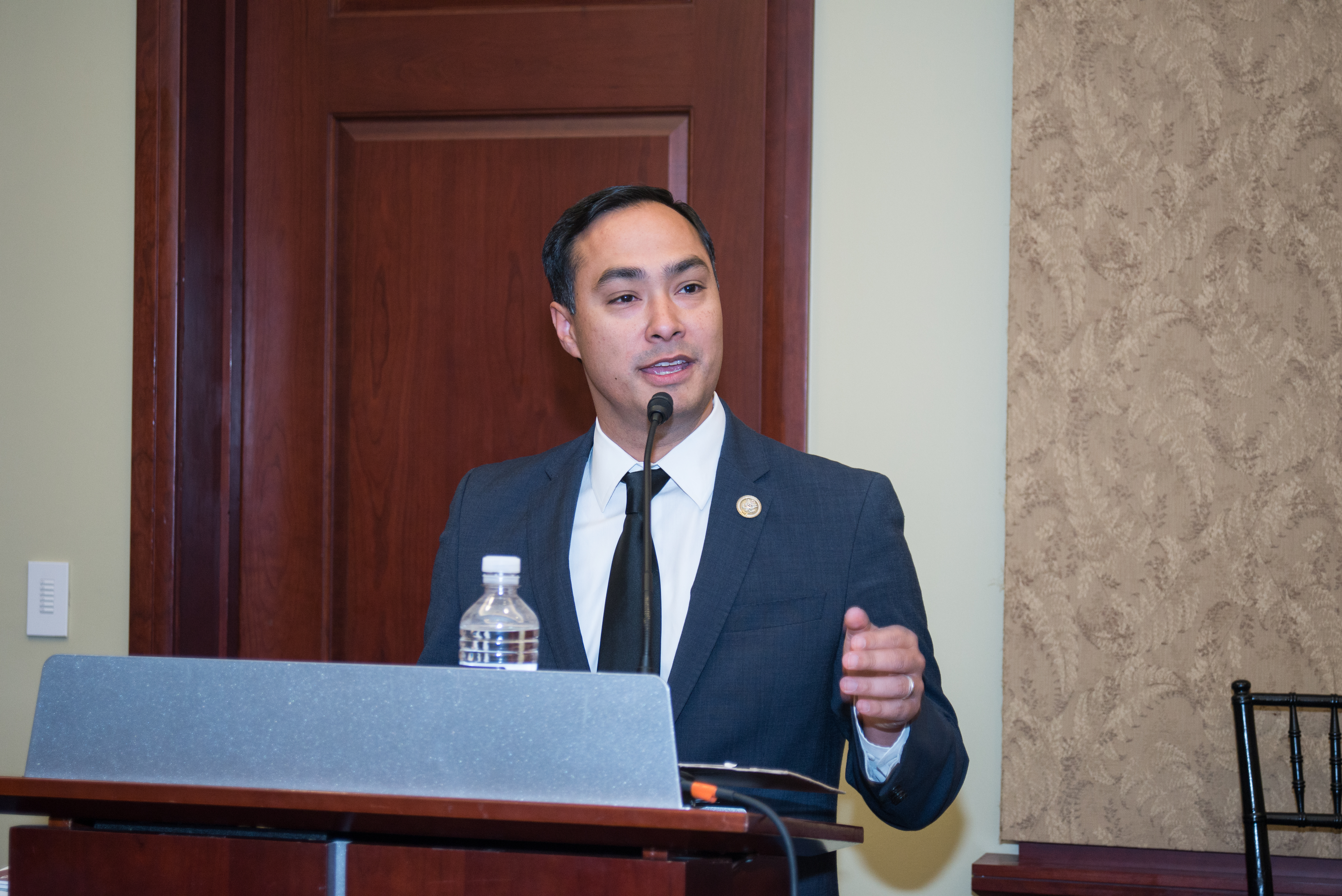The image captures an Asian man, possibly a politician, speaking passionately at a podium. Dressed in a blue suit with a black tie and a round gold pin on his left lapel, he is gesturing with his left hand while addressing an unseen audience. The podium, made of wood, has a bottled water and a black microphone positioned in front of him. Behind him, there is a stark white wall with a brown corkboard and a dark mahogany door. The setting appears to be a formal or political speaking event, and the composition, while professional in tone, could be the work of an amateur photographer. The colors in the photograph include shades of reddish-brown, tan, peach, black, white, gray, blue, and possibly dark green.